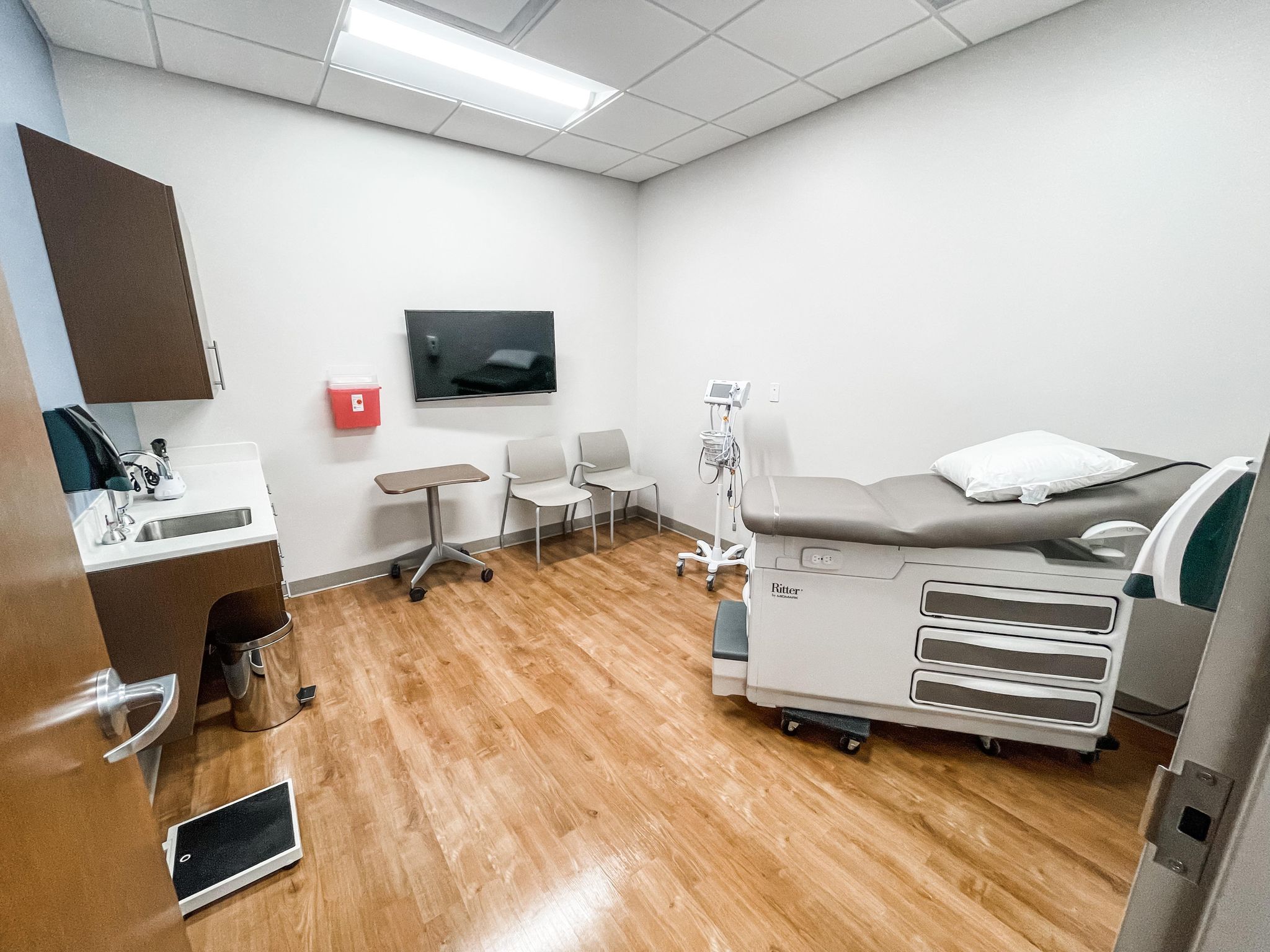The image depicts a detailed view of a clean and organized doctor's office from the perspective of someone standing in the doorway. Dominating the right-center of the room is an examination bed with a white cushion and pillow, resting atop a large white pedestal, designed for electronic adjustments. The floor is covered in polished, light-colored hardwood that gleams under the typical fluorescent lighting.

On the far wall, a flat-screen TV is mounted, approximately 40 inches in size, positioned slightly off-center to the right. Below it, there are a couple of gray chairs neatly arranged, and a mobile medical tray with four caster wheels stands close by. To the left of the TV, a red biohazard container for safe needle disposal is prominently attached to the wall.

The left side of the room features a practical sink area with a white countertop and a shiny metal sink embedded in it. Above the counter is a brown cabinet, providing additional storage, and a towel dispenser is mounted nearby on the wall. Beneath the sink is a brown cabinet that blends tastefully with the rest of the decor. A metal garbage can and a floor scale are also present in this area, enhancing the room's functionality.

The walls are primarily white, providing a crisp, sterile ambiance, with one wall painted blue for a subtle contrast. The room is sparsely decorated, with no paintings or anatomical drawings, emphasizing its clinical purpose. The neat arrangement of medical equipment, including a blood pressure monitor on a stand with a display and accessory basket, further enhances the room's atmosphere as a well-prepared, professional medical environment.